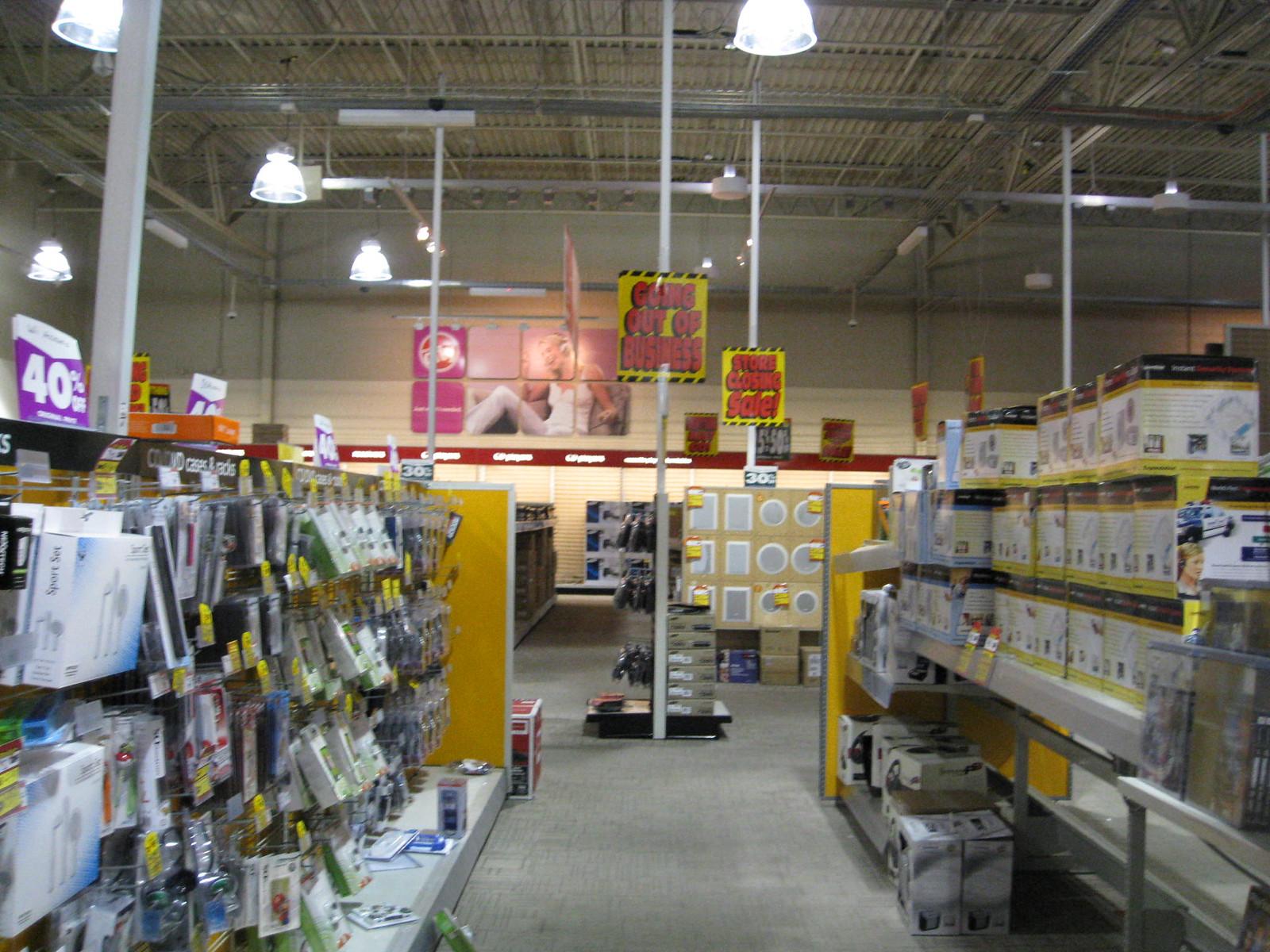The image depicts the interior of a large retail establishment with notably high ceilings, illuminated by long, bowl-shaped hanging lights that cast a white glow. The left side of the picture features an aisle stocked with electronic accessories displayed on various racks, while the right side mirrors this with more electronic accessories and a variety of small items neatly hanging on hooks. White boxes with black and gold accents, along with others featuring blue, are visible on the shelves. Dominating the top of the photo is a prominent sign with a yellow background and large red letters proclaiming "going out of business," accompanied by a "store closing sale" notice. In the background, a large poster shows a lady wearing a white shirt and pants, leaning back. Additional signs in the store highlight a "40% off" discount, underscoring that the store is in the midst of a significant liquidation sale.